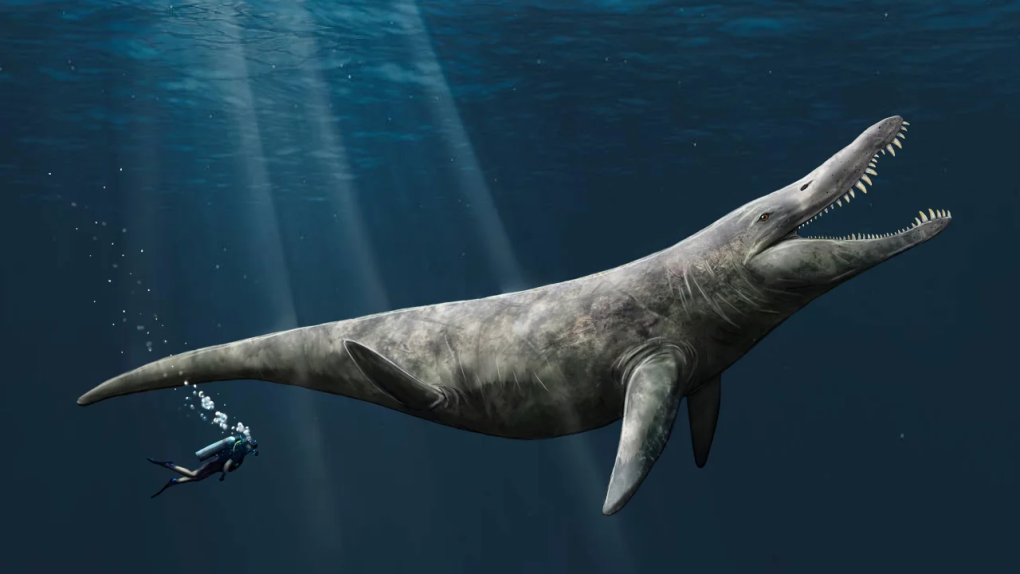This evocative image, seemingly an artist's rendition, plunges us into the depths of a prehistoric ocean. It showcases an extraordinary and colossal sea creature, poised mid-swim with its gaping mouth lined with serrated, razor-sharp teeth reminiscent of a shark, yet its immense body aligns more with that of a whale. This jaw-dropping creature measures over 100 feet in length, its mouth alone spanning 2 to 3 human lengths. The creature's form is accentuated by two sets of flippers, strategically placed one third and two-thirds down its body, leading to a thin, tapering tail.

The scene is bathed in a dim, deep blue light, with rays of sunlight piercing through the waves from the surface, creating a dramatic underwater landscape. A human diver, equipped with a single scuba tank on their back, adds a sense of scale and vulnerability to the tableau, as their tiny form—blowing a trail of bubbles upwards—approaches the gargantuan beast. The diver, not even the size of the creature's mouth, further emphasizes the monstrous proportions and ominous presence of this primeval leviathan. The dark, hauntingly beautiful backdrop of the deep ocean enhances the eerie and majestic ambiance of this fantastical tableau.